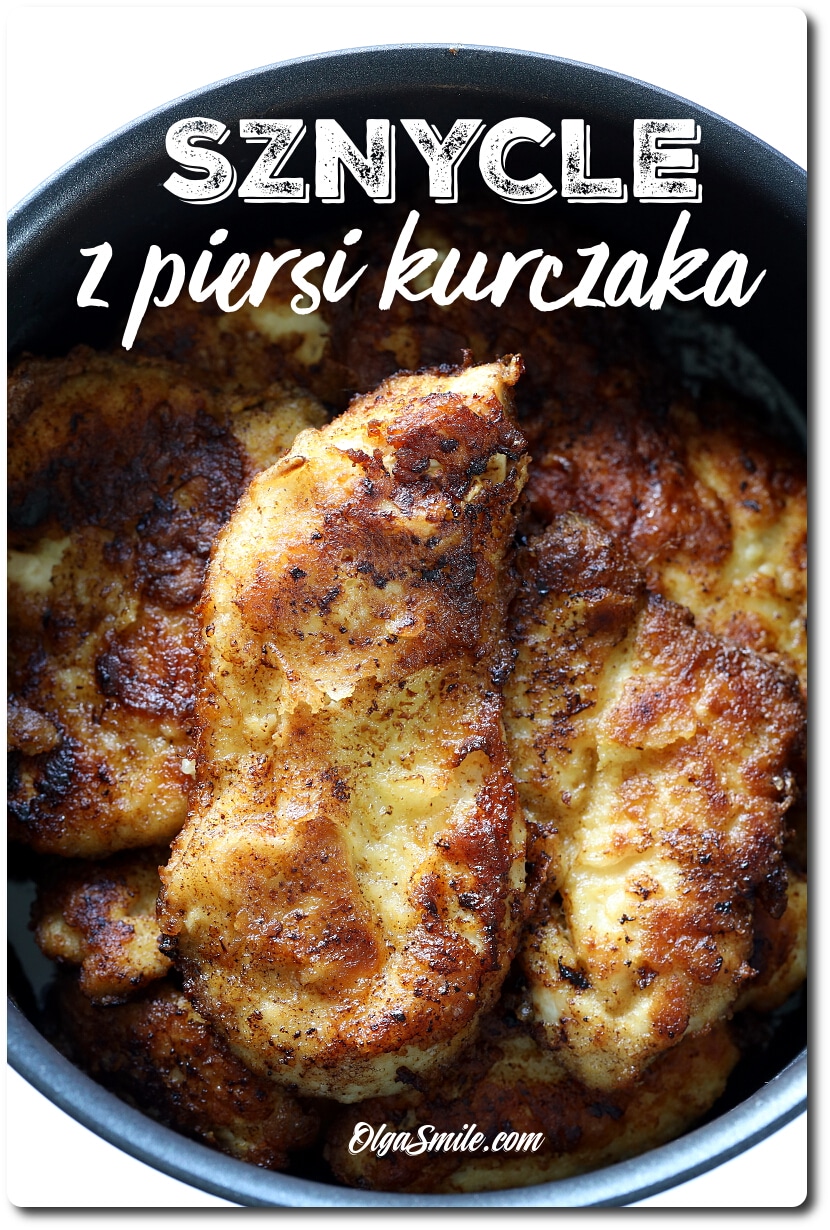The image showcases a close-up, top-down view of a black bowl filled with enticing, golden-brown chicken pieces, which appear to be grilled, fried, or baked. The chicken is sliced into numerous pieces and has a deliciously glazed appearance. The bowl contrasts sharply against the stark white background. At the top of the image, boldly written in dynamic, all-capital letters with a blocky, stencil-like font and a white drop shadow, is the word "SZNYCLE," which is followed by additional text in Polish—"Z PIERSI KURCZAKA." At the bottom of the image, the website "OlgaSmile.com" is written in a small, elegant brush script font, also in white. This image serves as either an advertisement or a menu option for the dish.